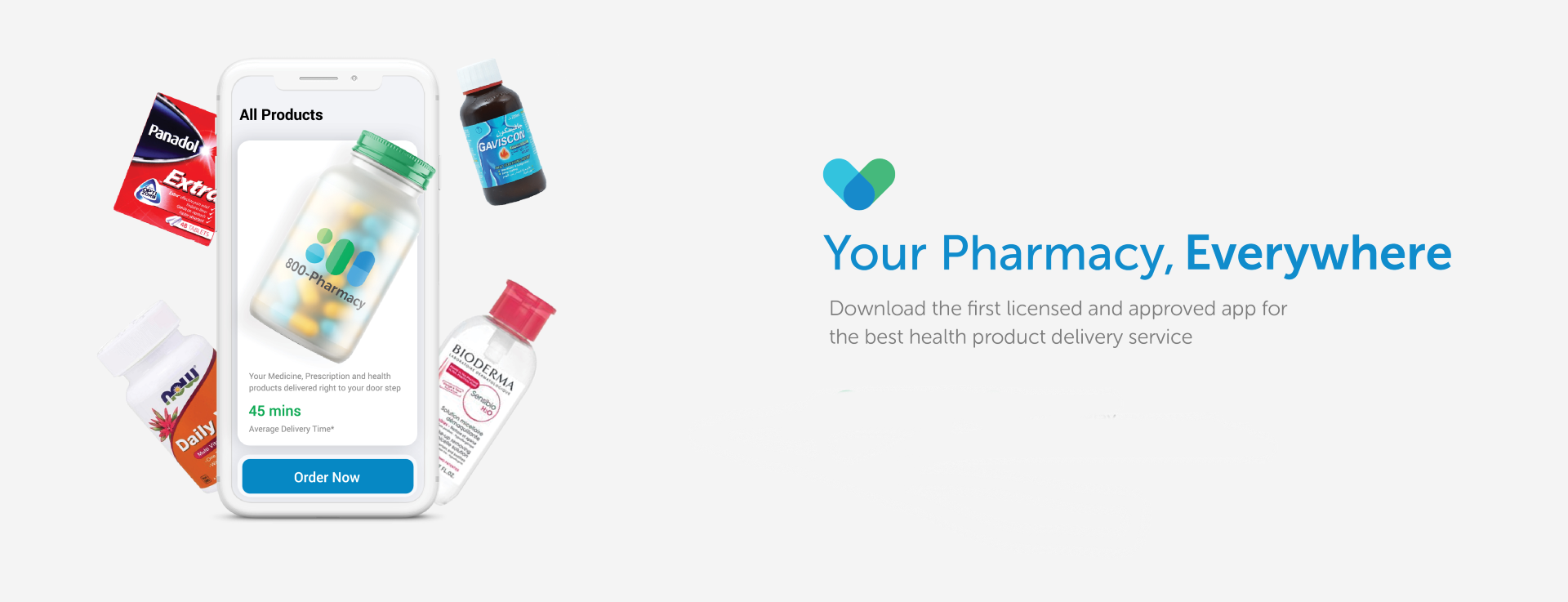The image appears to be an advertisement for a pharmacy delivery service. The background features a gray rectangle. On the left side of the image, there's a white smartphone displaying a phone case. The phone case shows the text "All Products" in black. Below that, there's an example product depicting a small bottle with a green cap labeled "800 Pharmacy." Additional readable text includes "45 minutes average delivery time" and a promotional tagline about having your medicine, prescription, and health products delivered directly to your front door. There’s also a prominent blue "Order Now" button.

Surrounding the phone, various products are displayed. In the top left corner, the brand "Panadol" is visible, followed by another text that begins with "Daily..." Underneath the text on the right side, the brand "Bioderma" is displayed next to a bottle. Adjacent to these elements, a blue and green symbol is presented with the phrase "Your Pharmacy Everywhere" in bold blue text. Below this, a small gray paragraph reads: "Download the first licensed and approved app for the best health product service delivery."